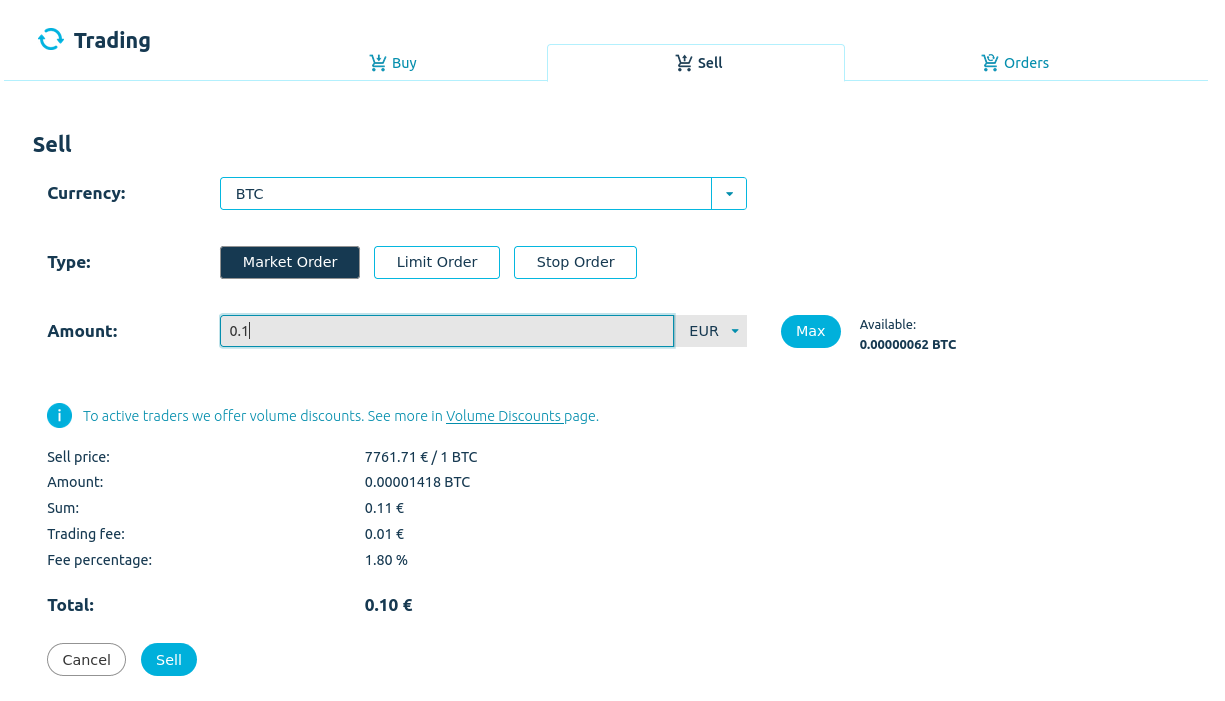Illustration of a comprehensive trading platform interface with an all-white background. In the center, on the right and left sides, blue arrows are strategically placed, one pointing left and curving into a circular formation with another arrow. This graphical element is situated about halfway down the frame.

To the right of this circular arrow graphic, the word "Trading" is prominently displayed in bold black text. Adjacent to it, in blue, is the label "Bligh" accompanied by a blue cart icon. Further to the right in black text is the word "Sell", followed by a black card icon. To the right of this, in blue text, is the word "Orders", also with a blue card icon. 

Directly beneath "Trading" in bold black text, another "Sell" is indicated, followed by the word "Currency". Below this is a long white rectangle with a blue border, containing the text "BTC" in black.

Moving downwards and towards the left, "Type" is displayed in bold. Under this, a blue tab with white text reads "Market Order". Adjacent to this tab are two white tabs with blue borders and black text, labeled "Limit Order" and "Stop Order".

Further down and to the left is the label "Amount" with a long grey rectangle beside it, showing "0.1". To its right, a blue tab with white text reads "Max". Below and back to the left again, there's a blue circle with a white lowercase "i" inside it, followed by a blue line providing additional information.

On the left side, further down, the interface lists several items: "Sell Price", "Amount", "Trading Fee", "Fee Percentage", and a bolded "Total". Corresponding numbers are displayed to the right of each label. 

In the bottom left corner, a white tab with a black border and black text reads "Cancel". Next to this, a blue tab with white text reads "Sell".